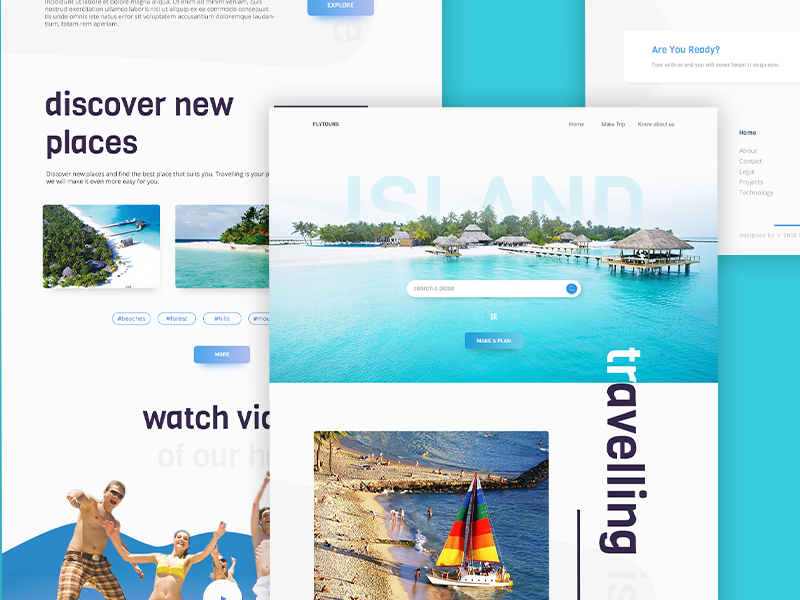This screenshot depicts a collage of various sections of a travel website. Dominating the center of the image is the top portion of the website, featuring a header with the logo 'Flytours' in the top left corner and navigation buttons labeled 'Home,' 'Make Trip,' and 'Know About Us' on the right. The main visual highlight at the top is a large, captivating photograph of a tropical island, complete with straw-roofed huts, a pier extending into clear blue water, and pristine white sand beaches. Situated beneath this idyllic image is a functional white search bar with the placeholder text "search a," accompanied by a prominent blue button labeled 'Make a Plan.'

The collage also includes two additional sections of the website, located to the left and right. On the left side, there is a segment titled 'Discover New Places,' which showcases several thumbnail images to inspire potential travelers. The right side of the collage is comprised of interface screens, further detailing the website's layout and design elements.